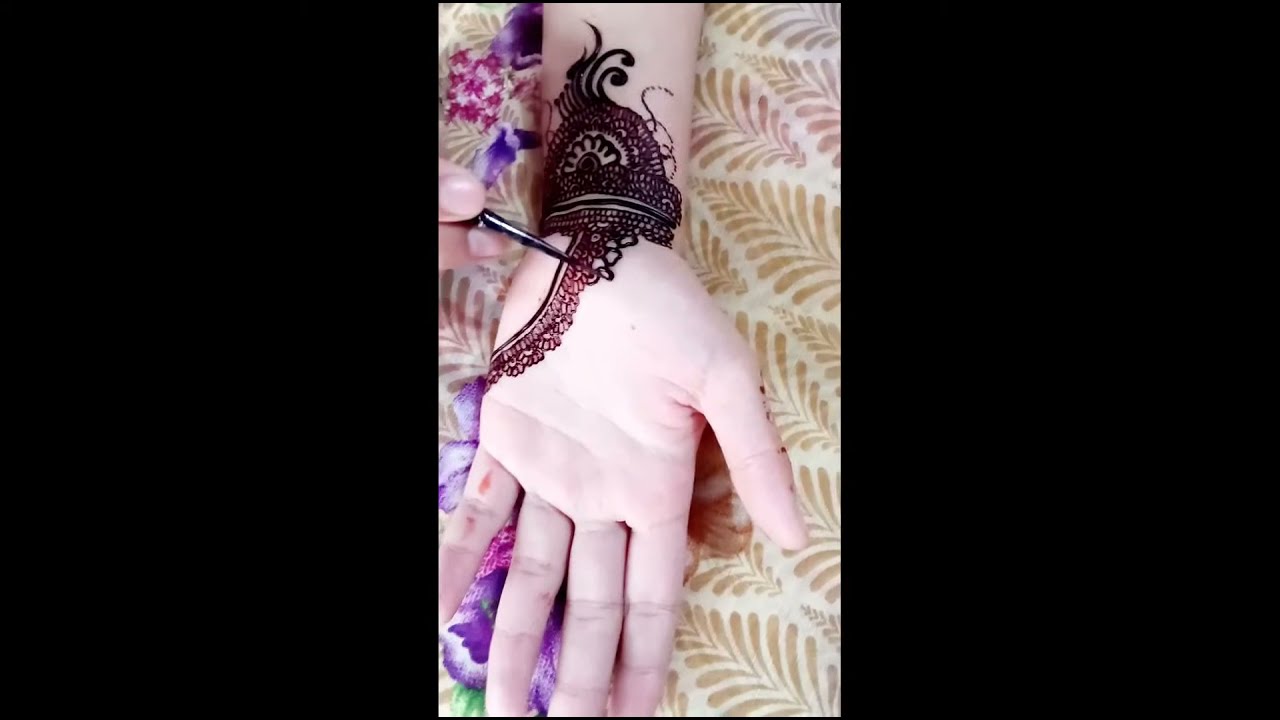A close-up photograph captures the artistic process of henna application on the palm and wrist of someone's left hand. The palm is facing upward with fingers pointing towards the viewer, and the wrist positioned at the top of the image. The intricate henna design starts from the wrist, extending over the palm, and features a lacy, floral pattern interspersed with small vines, curls, and circular details. The henna appears in dark brown, contrasting prominently against the person's lighter skin tone and enhancing the delicate intricacy of the design. The person holds a black applicator pen as they work on the bottom left part of their palm.

The scene is set against a fabric background adorned with a brown floral pattern, complemented by purple and pink leaves. Additional elements such as yellow and red trees are subtly visible, enriching the colorful backdrop. The detailed henna art, reminiscent of a series of bracelets and lace arches, stands out vividly, reflecting the meticulous craftsmanship behind it.